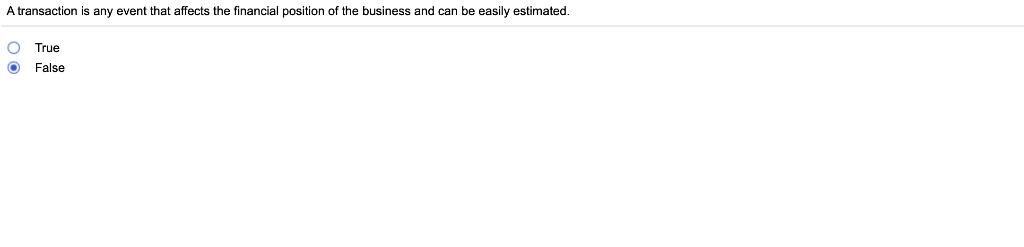This screenshot captures a detailed view of a single question from an online exam. The question, written in small black font, reads: "A transaction is any event that affects the financial position of the business and can be easily estimated." A thin grey line runs horizontally underneath the question, spanning the width of the screenshot. Below this line, aligned to the left, are two answer options labeled "True" and "False," each accompanied by a circular click bubble. The "False" option is visibly selected. The remainder of the screenshot appears blank, emphasizing the single question displayed with its answer choices in small black text.